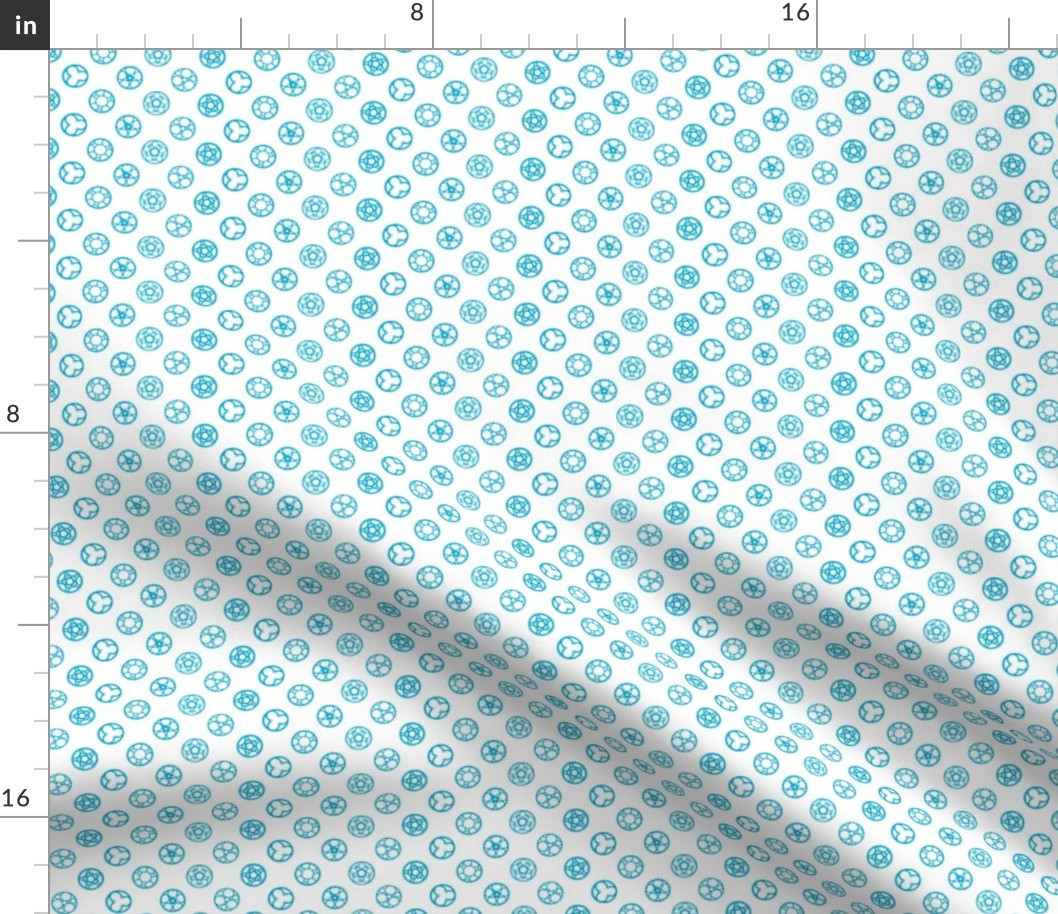This photograph captures a fabric swatch meticulously placed against a white background, showcasing its intricate pattern and measurements. The swatch, measuring approximately 21 by 18 inches, features a repetitive array of teal circles, each about half an inch in diameter. Despite being uniformly teal, the circles are adorned with varied internal shapes, including pentagrams, triangular patterns, and wheel-like designs, lending a complex yet unified aesthetic to the fabric. Along the top and left edges of the image, a ruler printed in black clearly marks inch measurements, with notable indicators like the numbers 8 and 16. The simplicity of the white and teal color scheme contrasts with the busy, detailed symbols within the circles, offering a visually engaging textile perfect for sewing or crafting projects.